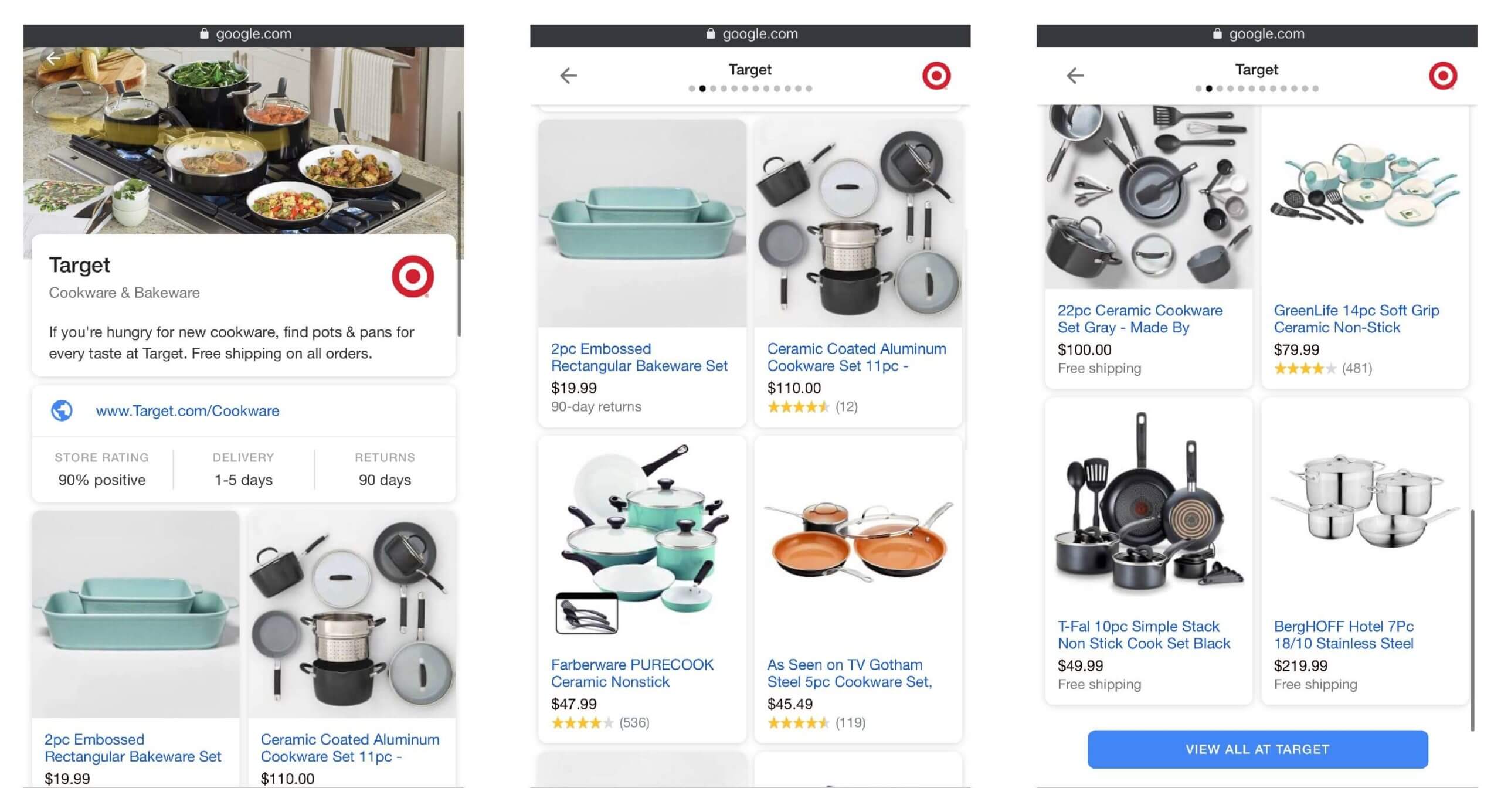A detailed screenshot from the Target website showcases a wide variety of cookware and bakeware options available for purchase. At the top left corner, a black border displays "google.com". Below, a stovetop brimming with pots filled with food sets an inviting scene.

On the left side of the screen, the text "Target Cookware and Bakeware" appears against a white background. The following promotion entices customers, "If you're hungry for new cookware, find pots and pans for every taste at Target. Free shipping on all orders." The iconic Target bullseye logo is prominently displayed in red and white circles. 

Further down, www.target.com is highlighted in blue text followed by details emphasizing a positive store rating of 90%, delivery timeframes of one to five days, and a 90-day return policy. Two product images are displayed: a two-piece embossed rectangular bakeware set in turquoise priced at $19.99, and an 11-piece ceramic-coated aluminum cookware set in black and stainless steel available for under $10. 

On the right, under the recurring "Target" header, multiple pages are indicated by little dots adorned with the Target bullseye. The same two products previously mentioned are shown again, alongside additional offerings including:

- "Farberware Pure Cook ceramic nonstick" at $47.99.
- "As seen on TV Gotham Steel five-piece cookware set" at $45.49.
- A "22-piece ceramic cookware set in gray" priced at $100 with free shipping.
- "Green Life 14-piece soft grip ceramic nonstick" for $79.99 with an accompanying four-star gold rating.
- "T-Fal 10-piece simple stack nonstick cookware set in black" at $49.99 with free shipping.
- "Berghoff Hotel seven-piece 18/10 stainless steel cookware set" for $219.99 with free shipping.

At the bottom of the screen is a blue banner offering a convenient "View all at Target" option.